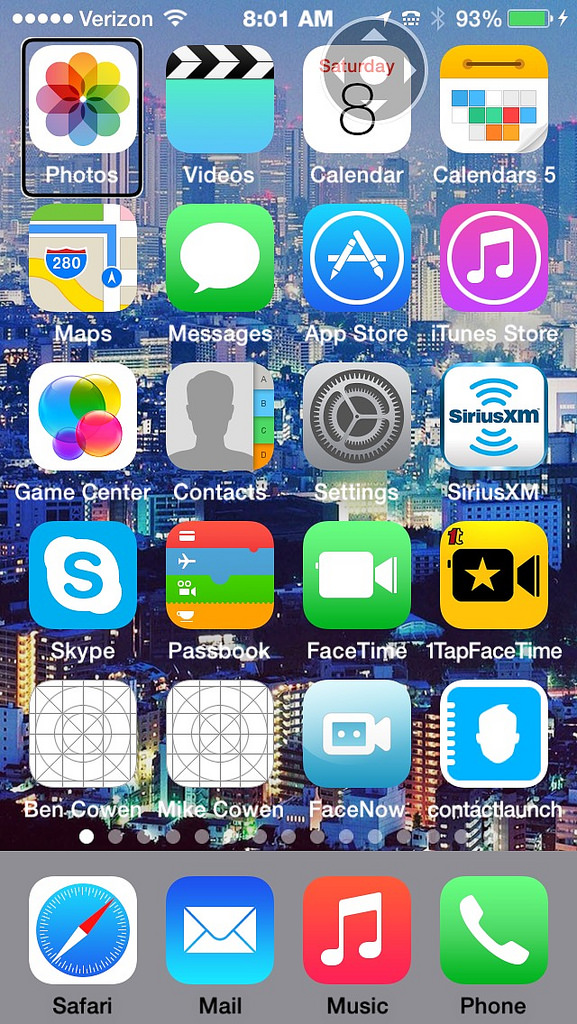The image displays the home screen of an iPhone. The status bar at the top indicates that the device is connected to Verizon's network and to the internet. The time shown is 8:01 AM, the battery is at 93%, and Bluetooth is active. The home screen features a variety of apps, including Calendar, Videos, Photos, Maps, Messages, App Store, iTunes Store, Game Center, Contacts, Settings, Sirius, Skype, Passbook, FaceTime, Contact Launch, Facebook, FaceNail, and personalized contact icons for Mike Cohen and Ben Cohen. Positioned at the bottom dock are the essential apps: Safari, Mail, Music, and Phone. The background wallpaper appears to be an image of a city skyline, although it is partially obscured by the numerous app icons prominently displayed on the screen.